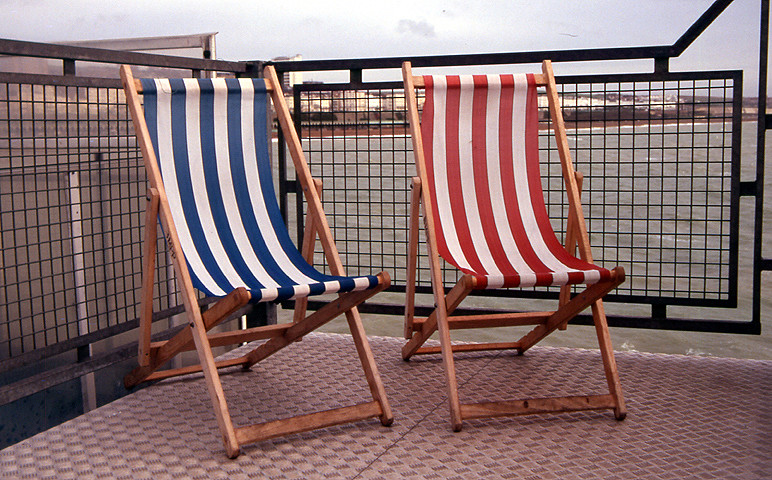The image is a detailed color photograph of two foldable sling-style deck chairs positioned on a balcony. Both chairs have light brown teak wood frames designed to fold for easy storage. The chair on the left features a vertical blue and white striped fabric seat, while the chair on the right showcases a similar vertical red and white striped fabric seat. They are set on a balcony with a geometric-patterned textured floor, possibly metallic. A black metal railing with window-pane patterned inset panels frames the background. Beyond this railing, a body of ocean water stretches out, suggesting the balcony is part of an elevated structure like a condo building, providing a panoramic view. Across the water, less than a mile away, are low-rise buildings, likely part of a beach town, under an open sky.